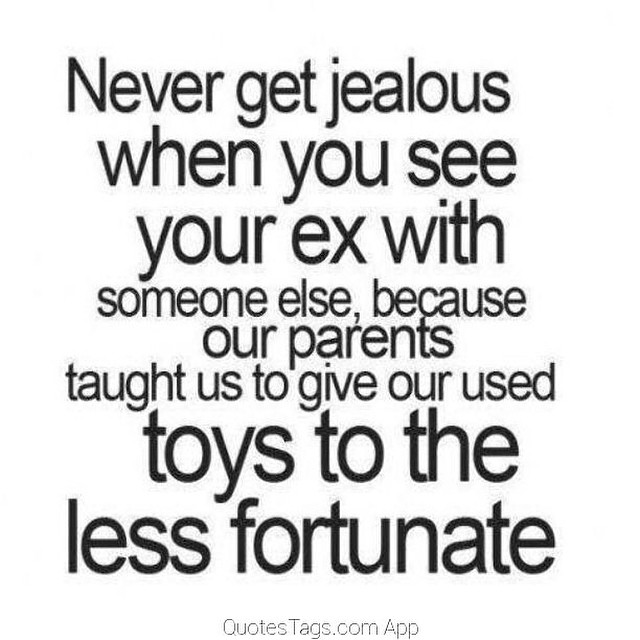The image is a humorous meme set against a plain white background, featuring various sizes of bold, black text. At the top are three prominent lines that read, "Never get jealous when you see your ex with," followed by a smaller line, "someone else, because," in medium black print. The next line, in larger black print, states, "our parents," followed by smaller text continuing the phrase, "taught us to give our used." The final part of the message in heavy black print reads, "toys to the less fortunate." Beneath the main text, a thinner, gray font notes the source as "Quotetags.com app." The meme humorously advises not to be envious of an ex, likening them to a used toy given to the less fortunate as per parental teaching.